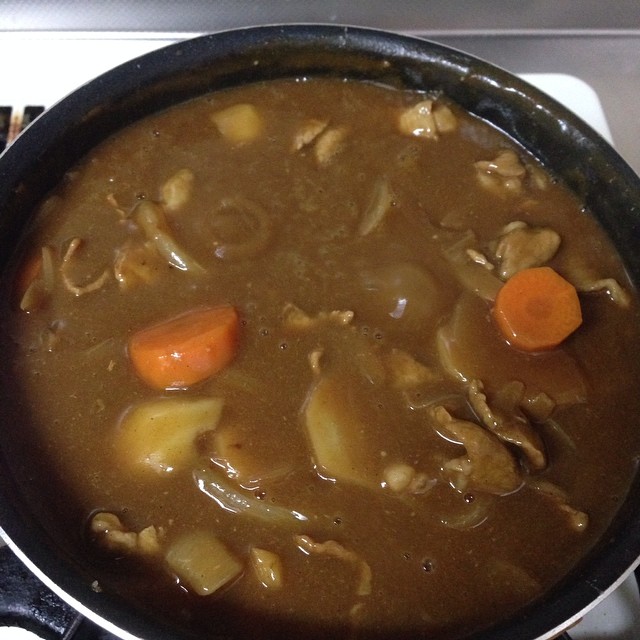The photograph captures a close-up view of a pot of hearty soup, nearly filling the entire frame. The soup is contained in a round black pot that features a silver or white rim, and it rests on a white stove surface with a grate in the background. The soup base is a rich, dark brown liquid, suggesting a thick, flavorful broth. Visible ingredients include prominently sliced round orange carrots, bits of light yellow potatoes, and white onions. There are also stringy pieces that could be noodles or small cuts of meat, with the possibility of some chopped vegetables adding to the texture and color. The soup appears slightly bubbly, indicating it is hot and freshly cooked. The composition suggests a cozy, home-cooked meal setting, likely prepared in a kitchen.